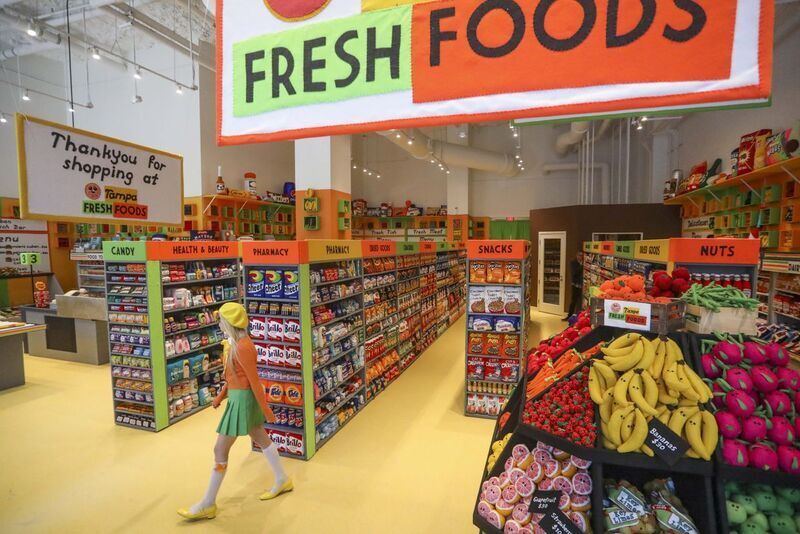This detailed color photograph captures the bustling interior of a Tampa Fresh Foods grocery store. Dominating the foreground on the left is a young woman with blonde hair, adorned in a distinctive yellow beret and an orange long-sleeve cardigan. Her outfit is completed by a pleated lime green skirt, white knee-high socks, and striking yellow Mary Jane shoes. She is walking toward the left end of the aisles.

The floor of the store is a vibrant yellow, and to the woman's right, one can see a produce rack laden with bananas, grapefruit, and other fruits. The store is neatly organized with clearly labeled aisles arranged in a row. The aisle markers indicate sections for candies, health and beauty, pharmaceuticals, snacks, and nuts, displaying black text against either red or green backgrounds. 

Overhead, a prominent banner stretches across the ceiling with parts that are green, orange, and white, featuring the word "Fresh" in black text on a green rectangular background and "Foods" in black text on an orange rectangular background. Nearby, on the left side of the image, another sign with yellow edges reads, "Thank you for shopping at Tampa Fresh Foods," accompanied by a smiley face to the left of the text. The store's ceiling reveals white-painted walls and visible piping, contributing to the open, airy feel of the space.